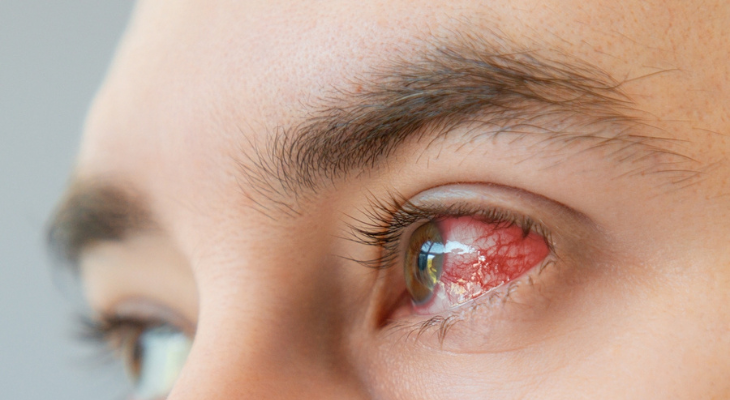This close-up photograph captures the upper part of a person's face, focusing primarily on their left eye, which appears severely bloodshot and inflamed, suggesting a possible infection or injury. The eye is dominated by visible red veins, and the white of the eye has a pronounced pinkish hue. The iris has a hazel coloration with a mix of greenish and brown tones. The person's eyebrow is brown and thick, and their eyelashes are relatively prominent. The right eye is partially visible in the background, looking healthy and normal with a clear white sclera. The image also shows part of the individual's nose and septum, and the triangular composition extends from the eyebrows to the upper part of the nose. The photograph is a horizontal rectangle with a gray background on the left side, emphasizing the contrast with the vivid details of the face.